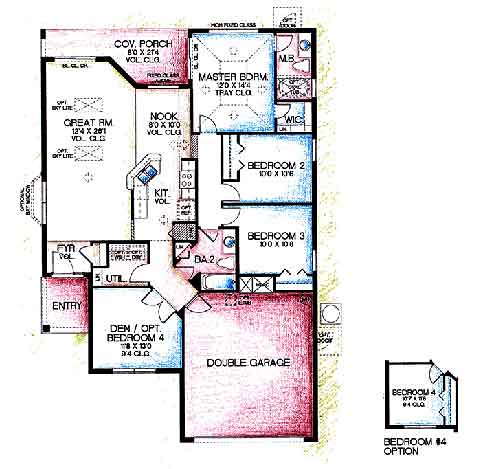This detailed architectural plan illustrates a three-bedroom house laid out in a basically rectangular shape. Starting from the bottom and moving upwards, the left side of the plan begins with a stairway structure. Adjacent to this, on the right-hand side, is a double garage, shown in red. Surrounding the house, particularly on the right-hand side, light green spotted coloring indicates areas designated for grass or brush.

Next to the double garage is a square labeled "Den/Opt. Bedroom 4," although its dimensions are not legible in the image. The entryway to the house is situated to the left of this area, marked in red.

On the lower right corner of the plan lies Bedroom #3, shaded in light blue and measuring approximately 10 feet by 10.8 feet, with a door opening into it. Adjacent to Bedroom #3, on the left-hand side, is a bathroom that includes a toilet and a shower.

Above Bedroom #3 is Bedroom #2, which measures about 10 feet by 13.8 feet. This space also features a door for entry and closet doors.

The top right-hand corner of the plan highlights the master bedroom, accompanied by a master bathroom, a water closet labeled "WIC," and a tub situated on the right-hand side. 

Toward the upper left of the plan lies a covered porch (COV Porch), measuring around 80 feet by 27.4 feet. Directly below this porch is a great room, denoted as "GRTRM," followed by a nook and finally, a kitchen located in the lower section of the house.

The plan also includes an optional configuration for a fourth bedroom, with separate notations detailing potential door configurations.

Overall, this house plan features multiple functional living spaces, optional flexibility for an additional bedroom, and clear distinctions for garage and outdoor areas.